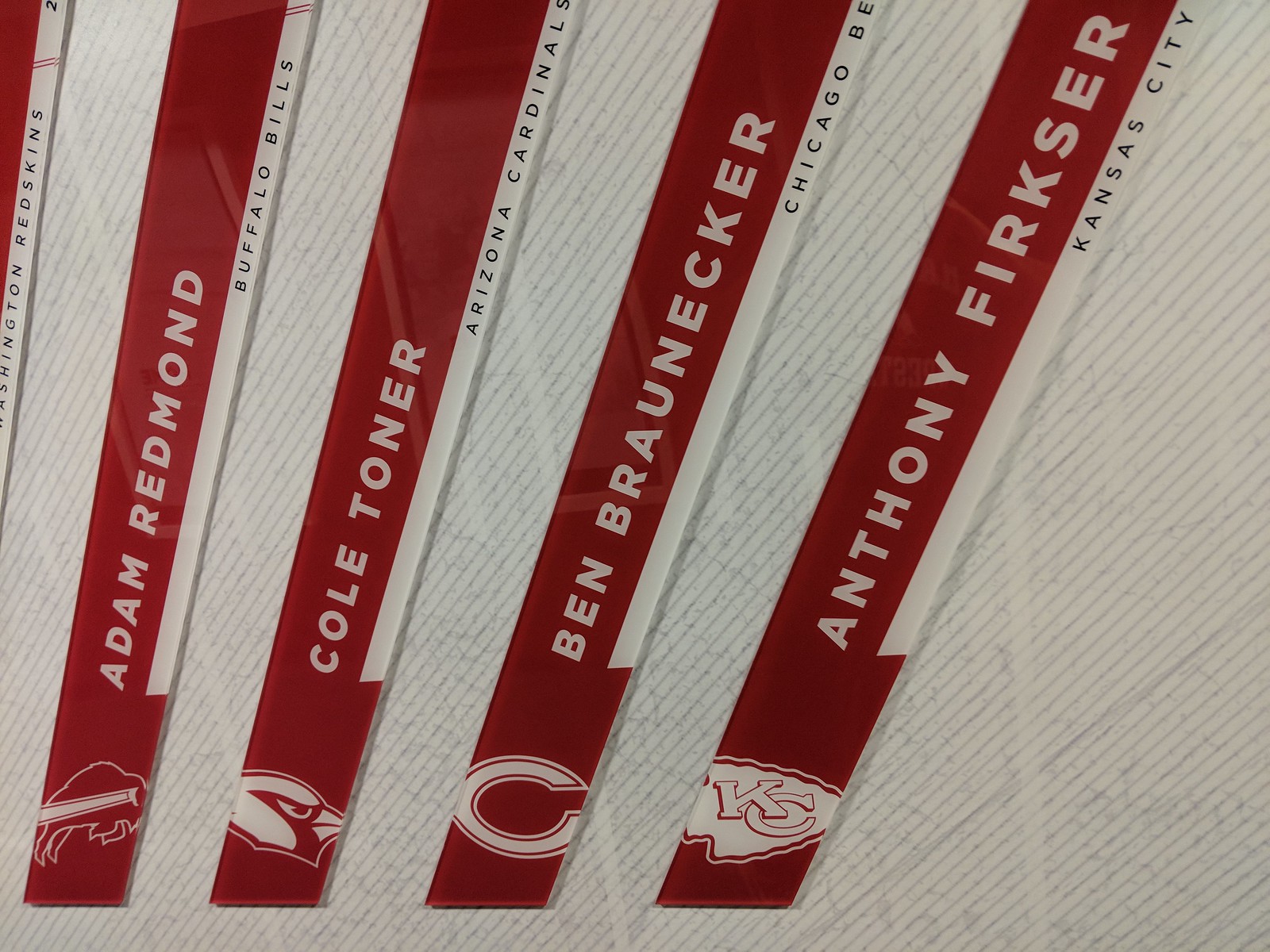This photograph showcases a series of vertically placed, elongated red banners against a white background adorned with thin diagonal gray lines. Each banner is meticulously arranged from top to bottom at a slight angle. Adorned at the top of each banner in white text are individual names and their respective NFL teams. The first banner displays "Adam Redmond" paired with the Buffalo Bills logo and name; the second banner reads "Cole Toner" with the Arizona Cardinals logo and name; the third banner shows "Ben Broniker" alongside the Chicago Bears logo and name; and the fourth banner features "Anthony Fersker" accompanied by the Kansas City Chiefs logo and name. Each banner consists of a white strip at the bottom with the team names written in black text next to their respective logos situated beneath. The combined elements of text, team symbols, and carefully placed banners create a visually captivating and organized display.